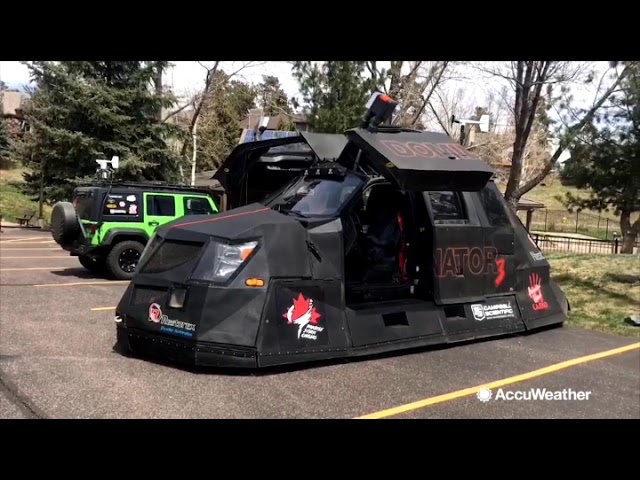This photograph, taken in a parking lot, features two vehicles and a background that fuses the mundane with the futuristic. In the forefront is a green Jeep Wrangler, notable for its vibrant lime green color and a mysterious white object on its roof. Adjacent to it is an enigmatic vehicle cloaked in a modified cover, imparting an appearance reminiscent of sci-fi and Ghostbusters aesthetics. This vehicle, possibly a modified SUV, features black coloring, red and white lettering, and what appears to say "Dominator" along its side, with unique suicide doors adding to its mysterious allure. The landscape is a typical suburban setting with hints of winter, as evidenced by the leafless variety of trees, pine trees, and patches of grass. In the distant background, a building is partially obscured. The image bears the "AccuWeather" watermark in its bottom right corner, suggesting a potential weather-related context for these visually striking vehicles.